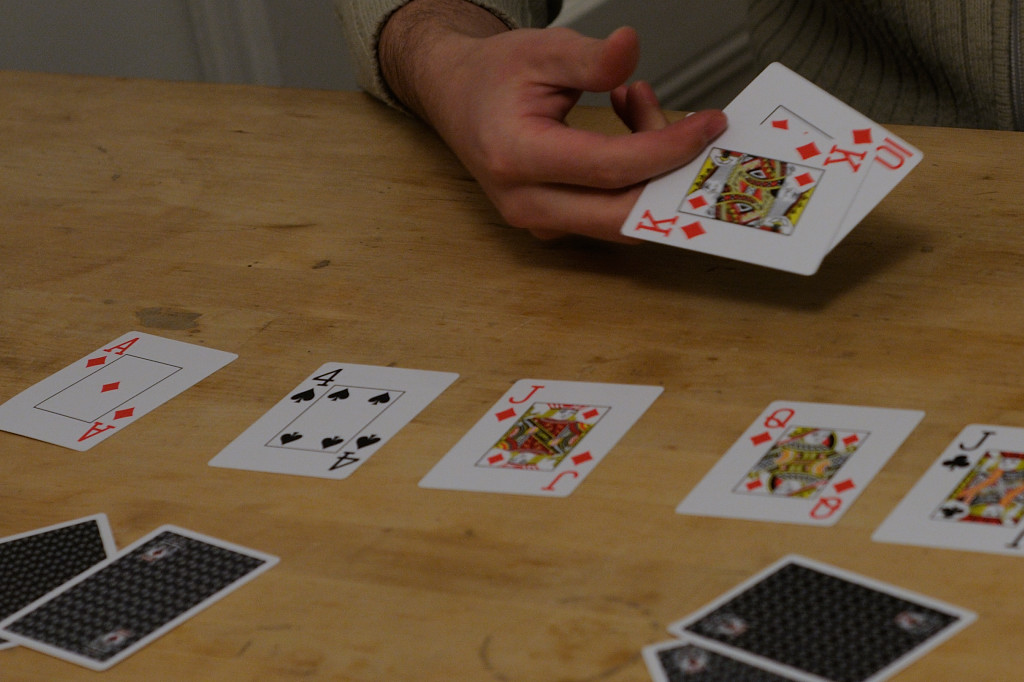The image captures a tense moment during a card game, focusing on a single player's hand and arm, partially obscured by the sleeve of their shirt. One hand clutches two cards: the King of Diamonds and the Ten of Diamonds. The setting is a well-worn brown wooden table, scarred with ring marks from past drinks. Laid out meticulously in front of the player are five cards—starting from the left: the Ace of Diamonds, the Four of Spades, the Jack of Diamonds, the Queen of Diamonds, and the Jack of Clubs. Two sets of cards lie face down—one pair opposite the Ace of Diamonds and the Four of Spades, and another set in front of the Queen of Diamonds and the Jack of Clubs—adding an element of mystery to the game. The background is minimalist, revealing only a small section of a white wall, directing all attention to the drama unfolding on the table.